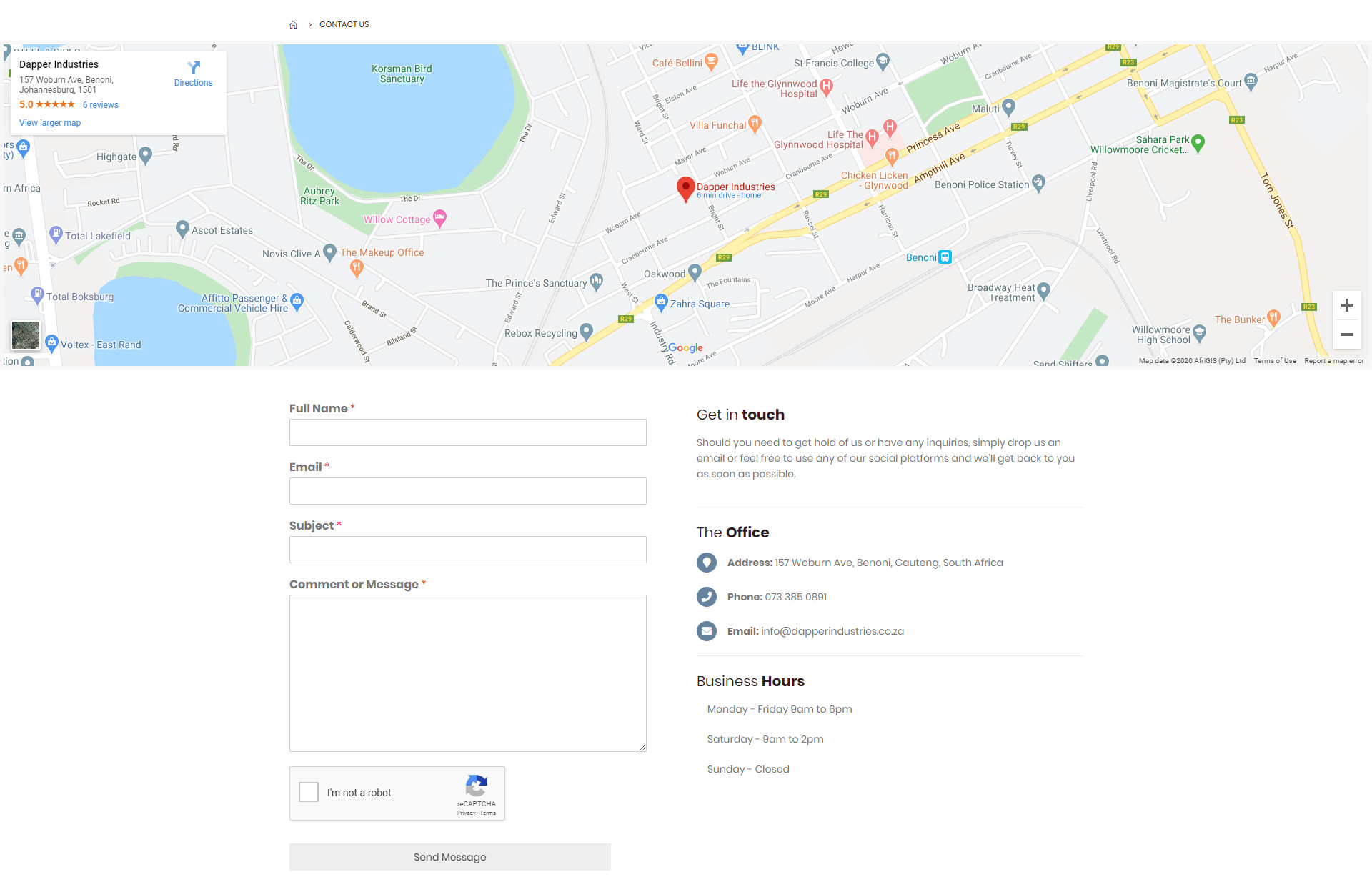This is a detailed caption:

The image is a screenshot of the contact page of Dapper Industries' website. The top left section features an embedded Google Maps view highlighting the surrounding area of the company's location. The top left corner of this map section displays the company's name, "Dapper Industries," followed by the address: 157 Wilbur Avenue, Benoni, Johannesburg, 1501. Below the address, there is a link for directions, an indicator showing six reviews with a perfect 5.0-star rating, and a button labeled "View Larger Map."

The bottom half of the page includes a contact form containing fields for "Full Name," "Email," "Subject," and a text box for a "Comment or Message." Below the text boxes, there is an "I'm not a robot" CAPTCHA, which has not been checked, followed by a "Send Message" button.

To the right of the contact form, there is a "Get in Touch" section that invites users to drop an email or use social platforms for inquiries, promising a prompt response. Under this message, there are office details: the address, 157 Wilbur Avenue, Benoni, Gauteng, South Africa; the phone number, 073-385-0891; and the email address, info@dapperindustry.co.za. The business hours are also listed: Monday to Friday from 9:00 AM to 6:00 PM, Saturday from 9:00 AM to 2:00 PM, and closed on Sundays.